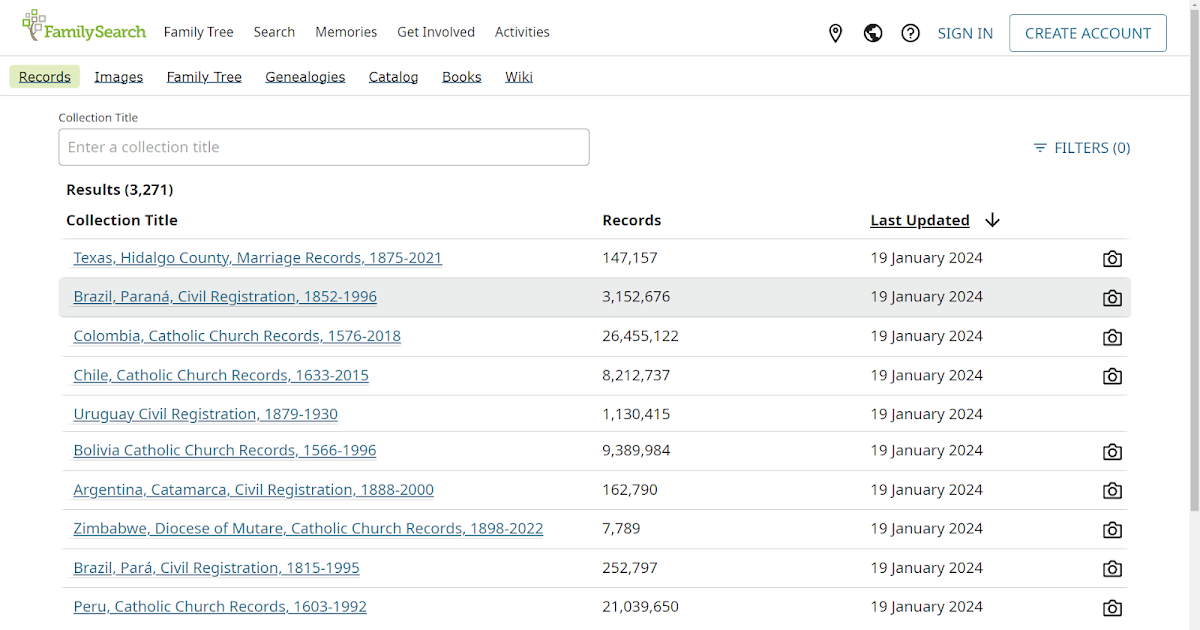The image is a detailed screenshot of the FamilySearch website interface. In the top left corner, the FamilySearch logo is prominently displayed, featuring the text "Family Search" in green alongside a tree icon composed of green and gray squares. To the right of the logo, the navigation bar offers multiple options including "Family Tree," "Search," "Memories," "Get Involved," and "Activities." Further to the right, "Sign In" and "Create Account" buttons are visible for user authentication.

Below the primary navigation bar is an additional set of navigational links within a green-bordered box. These options include "Records" (highlighted in green), "Images," "Family Tree," "Genealogies," "Catalog," "Books," and "Wiki." Directly underneath this navigation set is a search bar with the placeholder text "Enter a collection title," prompting users to search for specific collections by title.

The central area of the interface is dominated by search results. A heading indicates "3,271 results" found for the entered query. The results are organized into three columns: "Collection Title," "Records," and "Last Updated." Each row details a different collection. The first example is titled "Texas, Hidalgo County, Marriage Records, 1875-2021," with 147,157 records noted and a last update date of January 19, 2024. Each entry also includes a small camera icon to the right, implying the presence of image records. This structured format is consistent across all listed entries.